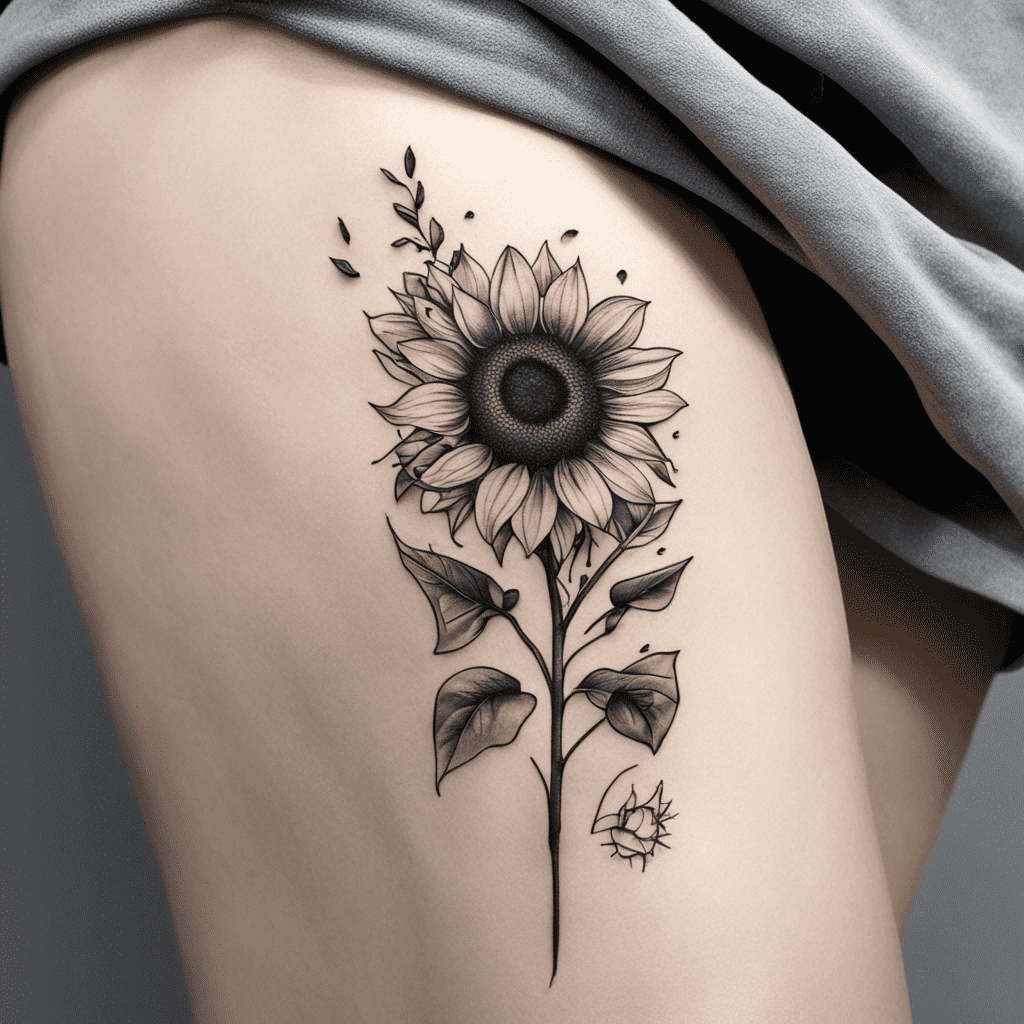The color image is a detailed close-up of a person's upper right thigh. The person, who has very pale skin, is draped in a soft gray fabric that is pulled up around the hip area, revealing the tattoo. The tattoo is a beautifully done black and white sunflower, prominently featured on their thigh. The sunflower has a dark center with numerous petals radiating outward. The stem extends downward and is adorned with leaves along its length, as well as a vine with additional leaves that wrap around the flower. At the bottom right corner of the tattoo, there is an unclear spiky design. The light gray background complements the soft gray fabric, making the intricate details of the tattoo stand out.